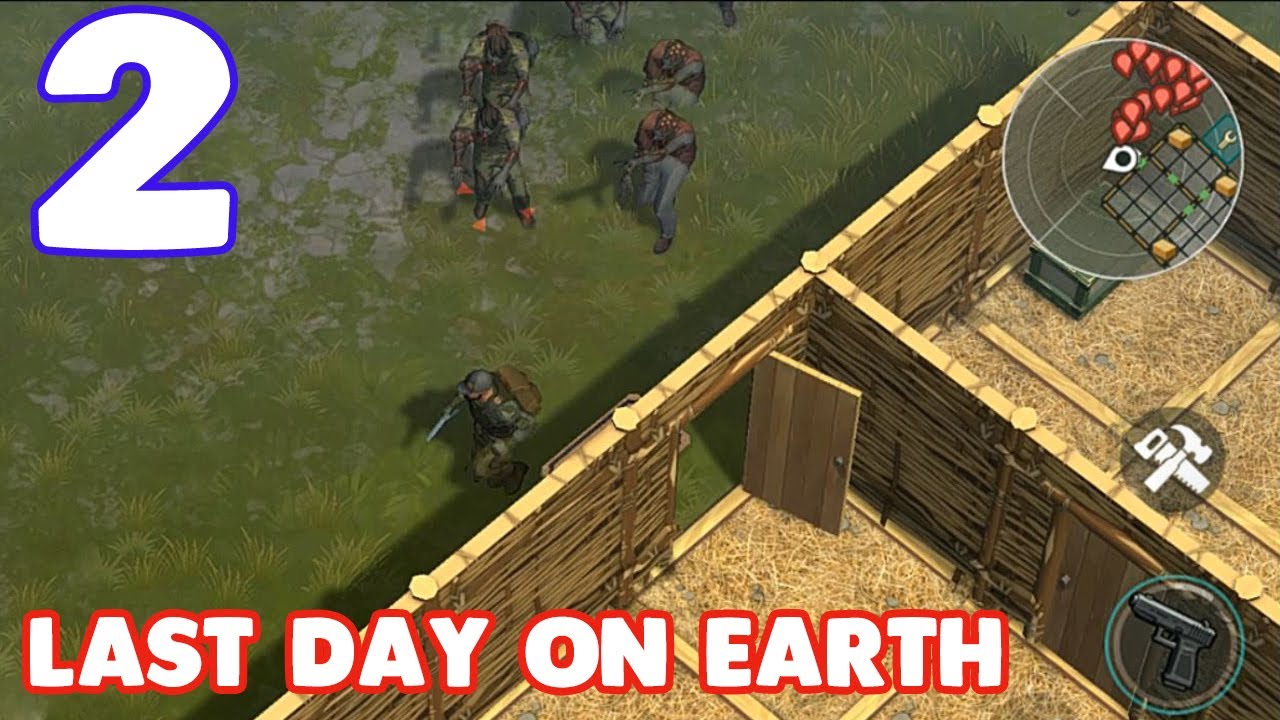This image is a screen capture from a video game, likely titled "Last Day on Earth." The display prominently features the game title in bold white letters outlined in red at the bottom. In the top left corner, a large white number "2" with a blue outline is visible. The scene is split diagonally between the exterior and interior of a rustic structure made from thatched wood and straw, with the left side showing an open door and the right side a closed one. Inside the building, there is a table and symbols of a hammer and saw, indicating possible tools for use in the game. Outside, a soldier in green fatigues and a backpack is being pursued by several zombies dressed in similar military gear. The bottom right corner shows icons of a revolver, likely the soldier's active weapon, and the aforementioned tools, which might be collectible items. The top right corner features a mini-map displaying the player's location and nearby targets.